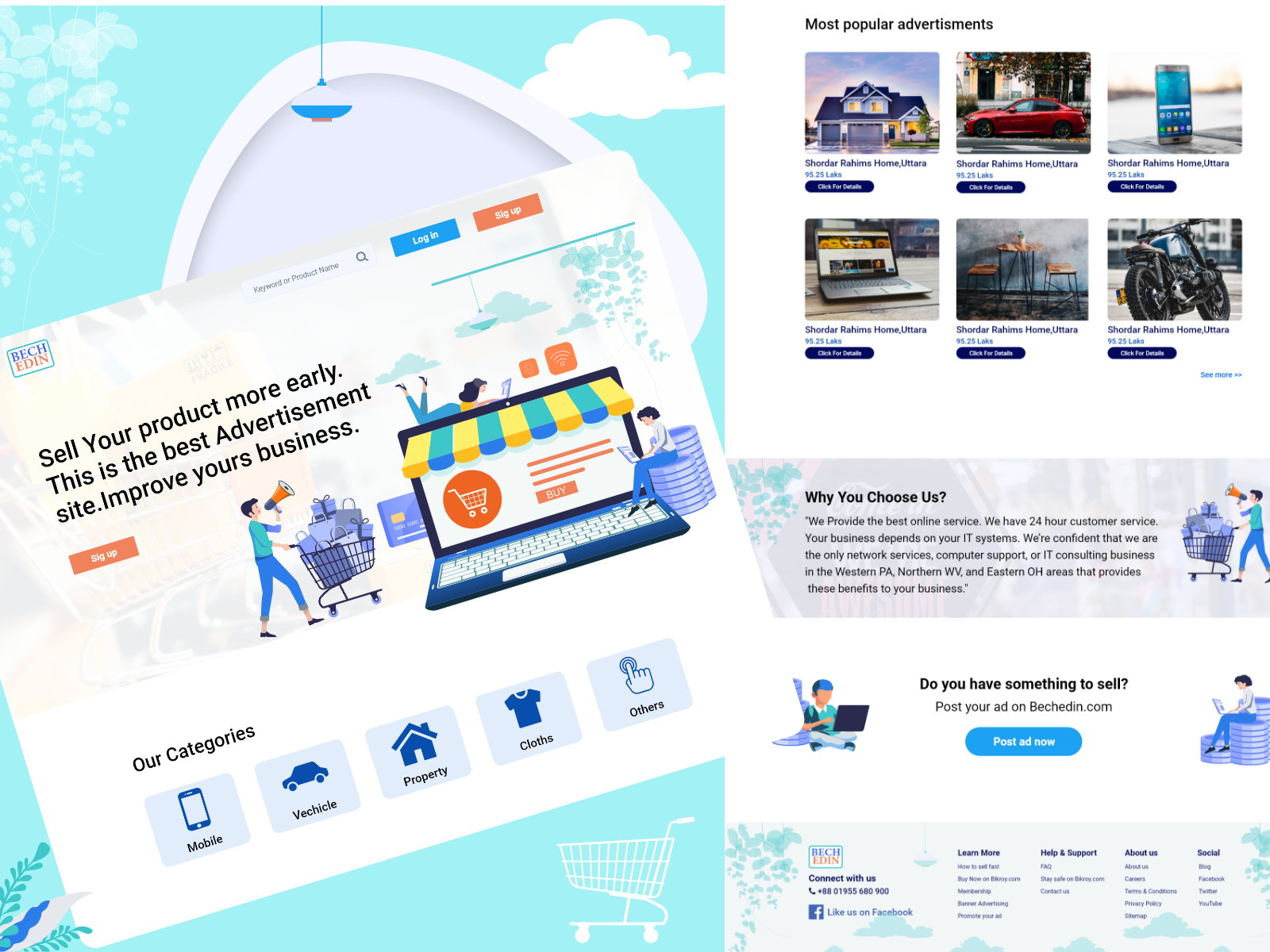The screen is divided into two distinct sections. The left section features a vibrant teal aqua blue background, housing a diagonally oriented screen displaying various pieces of information. Behind this screen is a unique white shape, resembling a circular triangle, with a small blue and white ball positioned at its apex. 

On the right section, the heading "Top Most Popular Advertisements" is prominently displayed. Below this heading, there are two rows, each containing three square images representing different advertisements. Beneath these images is a gray rectangular area featuring a section titled "Why You Choose Us," followed by a paragraph explaining the service's benefits. Further down, a white rectangle contains additional relevant information.

At the bottom of the right section, presumably, lies the site map of the webpage. This site map is placed on a light gray background with touches of turquoise print and hosts various clickable links.

Notably, the left section of the webpage includes an image of a person pushing a shopping cart. Additionally, there's a depiction of a laptop adorned with a storefront-like canopy, emphasizing an online shopping theme.